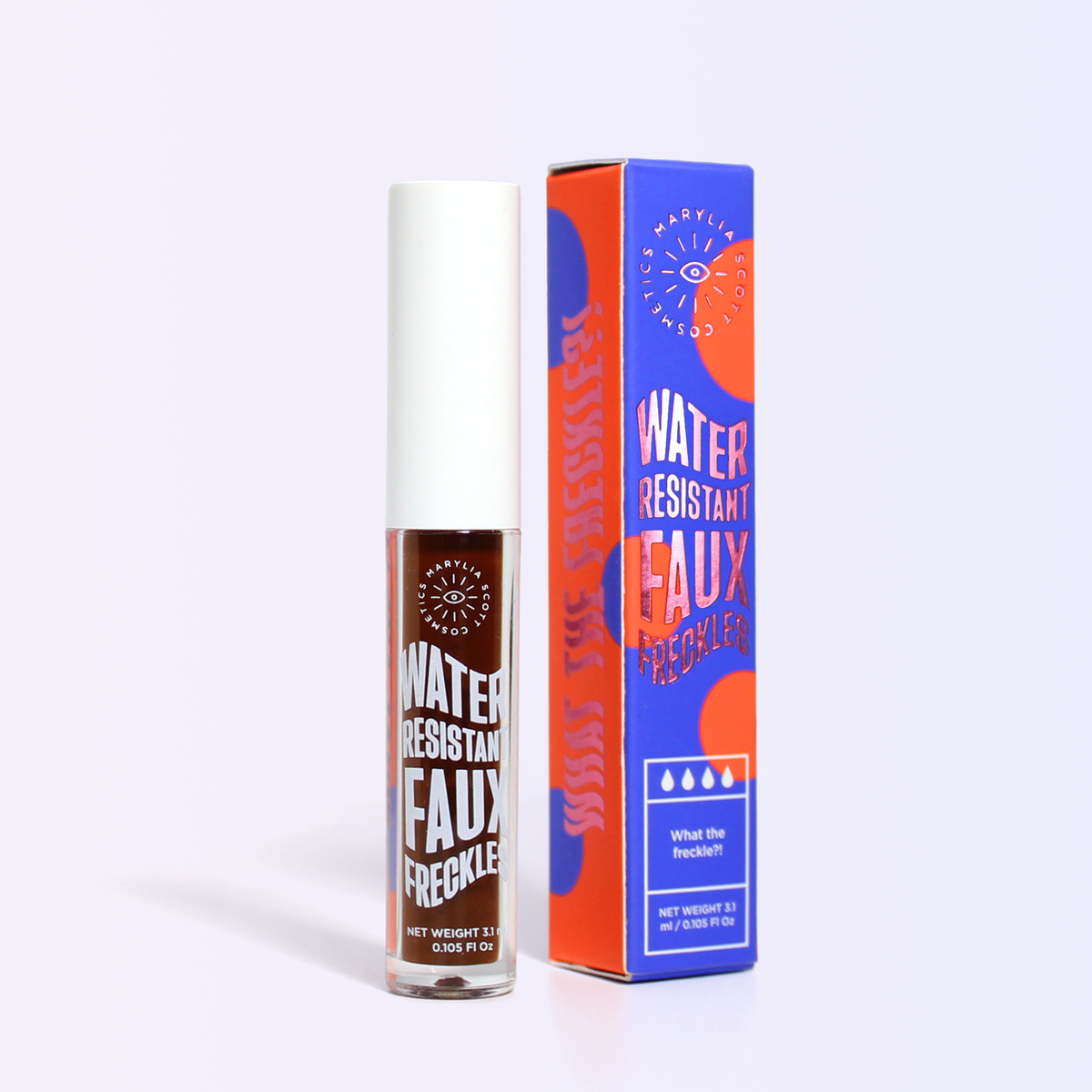This is a detailed color photograph of a cosmetic product, specifically an item of makeup. The photograph features both the product's jar and its packaging. The jar is a square glass bottle filled with a dark brown liquid, labeled with large, curvy white letters stating "Water Resistant Faux Freckles." The bottle is topped with an unusually long, white cap that appears to unscrew to reveal an applicator brush. Midway down the bottle, the Marilia Scott Cosmetics logo is visible, featuring an "I" with beams radiating from it and the words "Marilia Scott Cosmetics."

To the right of the jar is the product's packaging - a tall, vividly colored box. The box has a striking design with a blue background adorned with orange polka dots and silver lettering. Additionally, the side of the box is orange with blue polka dots. The front of the box prominently displays the same logo as the jar and repeats "Water Resistant Faux Freckles" in the same wavy, unique text style. At the bottom of the box, enclosed in a white section, are four droplets along with the phrase "What the Freckle!?" followed by the net weight of the product, 3.1 milliliters, or 0.105 fluid ounces. The side of the box also displays more text in silver, though it is not fully visible in the image. Overall, the photograph presents a vibrant and detailed view of this makeup item and its distinctive packaging.